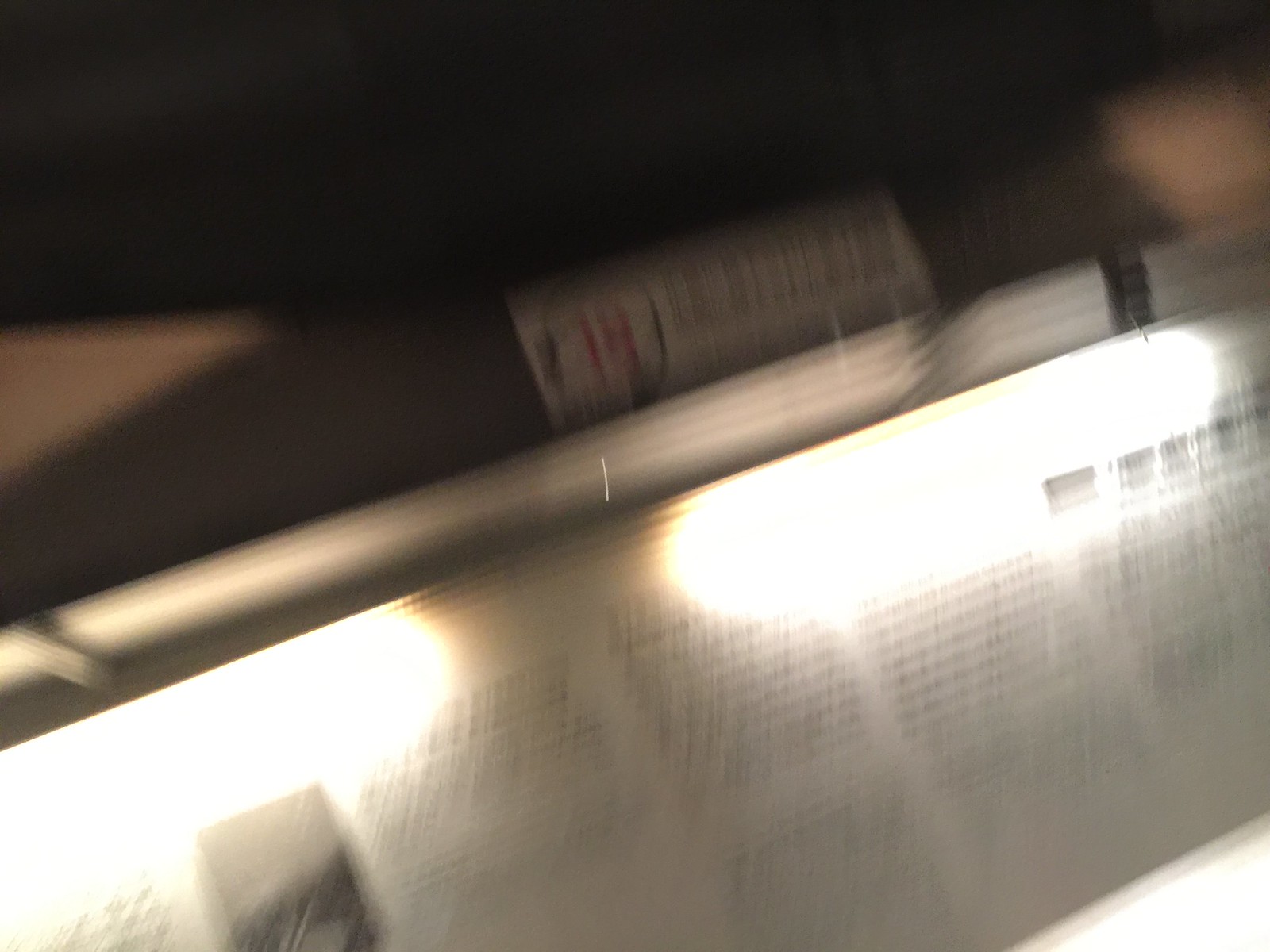A very blurry photograph captures a predominantly dark scene with a notably black top portion. From both the left and right edges of the image, a light source penetrates, illuminating parts of the scene. At the center, a white rectangular tab or label with black writing draws attention. Below this label, a prominent white bar stretches diagonally from the upper lower left corner to the upper right corner. Situated beneath the bar is an open newspaper or book, with reflections of bright light enhancing the left and right sides. The text in the image is black on a white background, with cursive writing visible. In the lower left corner, a small black and white picture can be seen, adding to the intrigue of the composition.